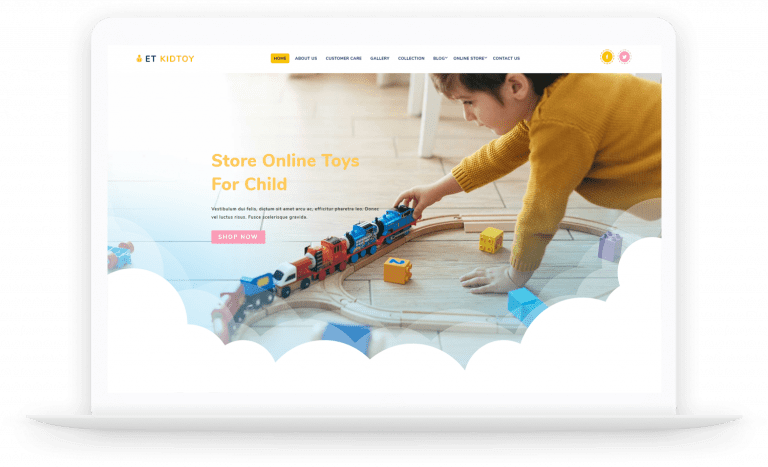This is a detailed screenshot of a webpage, likely displayed on a tablet or smartphone. The left-hand side features a white bezel on a gray background. Prominently displayed in black text is "ET," with "KID TOY" adjacent to it in bold orange letters. Towards the center of the webpage, there's a row of clickable buttons. The "Home" button is highlighted in orange, indicating it is selected, while the other buttons—labeled "About Us," "Customer Care," "Gallery," "Collections," an unreadable one, "Online Store," and "Contact Us"—are in black text and are unselected. The blurry button is likely "Blog."

On the far right, there is a circular icon with a floral and orange patterned border. The inner portion of the circle is orange with a white icon that appears to resemble an eye. To the right of this, there's a white bird centered on a pink background with a floral pink border, representing X, formerly known as Twitter.

To the right side of the screen, a child with short brown hair and light skin is playing with a train set. The child is wearing a mid-orange colored sweatshirt. The train set includes a blue and red train resembling Thomas the Train at the back, transitioning to a regular train at the front. Above the child in bold orange text, it reads "STORE ONLINE TOYS FOR CHILD." Below this, there is a pink button with the white text "SHOP NOW." The train track is wooden and brown in color.